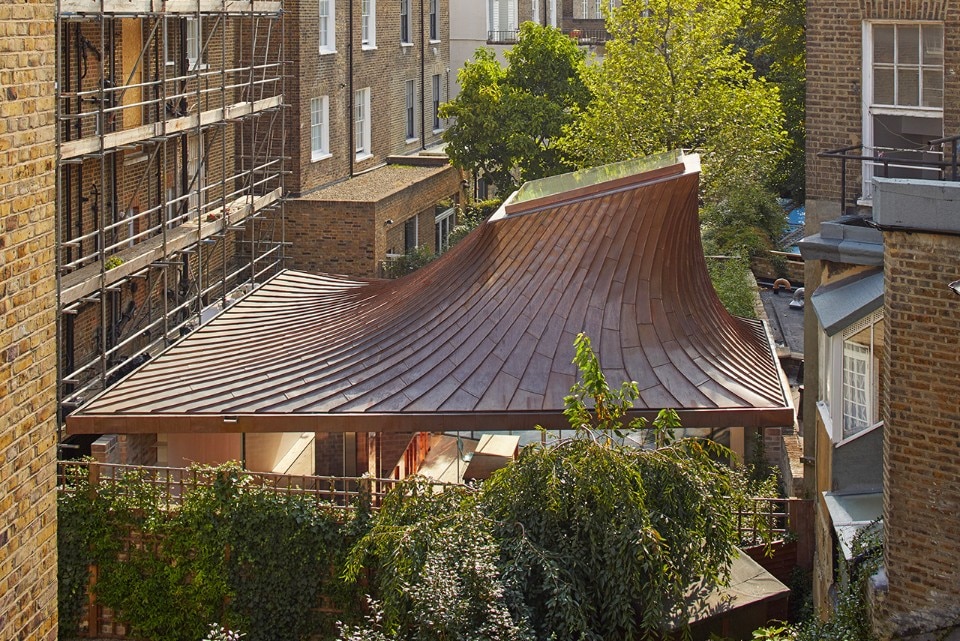This photograph, taken during a bright and sunny day, captures an outdoor setting featuring a unique and striking structure. At the center of the image stands a building with an unusual roof resembling a volcano, constructed with brown tiles that swirl upwards toward the top. Notably, the apex of the roof hosts a shiny and reflective solar panel. The roof serves as a canopy, sheltering an open courtyard area below. 

Surrounding this central structure are various buildings made of yellow, tan, and traditional red bricks, all adorned with numerous white window panes. On the left side, there is visible scaffolding on one of these buildings, hinting at ongoing construction or repairs. 

In addition to the architectural elements, the scene is enriched with lush greenery. Trees with vibrant green leaves flank the courtyard and some taller trees in the background, illuminated by the sunlight, add a bright contrast to the image. The combination of the eclectic architecture and verdant foliage creates a compelling and lively outdoor scene.